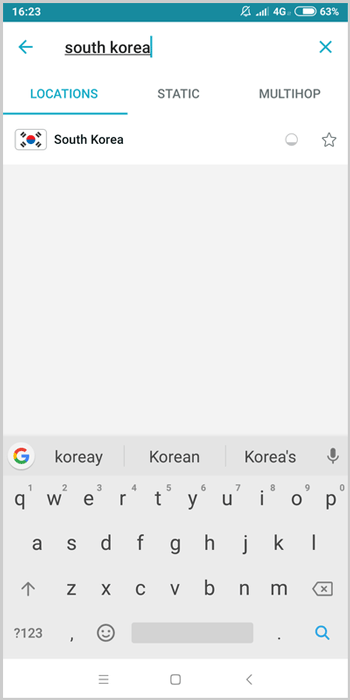**Descriptive Caption:**

This screenshot showcases the interface of a flight-search website accessed from a Samsung smartphone. The image has a white and grey background, with a light turquoise notification bar at the top displaying the time on the left and icons for battery percentage, no alerts, and cell phone signal on the right. Within the app, a search bar is positioned at the top where "South Korea" has been entered. Beneath the search bar, three options—Locations, Static, and Multi-hop—are available, with Locations currently selected. The search result displays "South Korea" accompanied by its national flag. Below the search result, there is a grey empty space. The smartphone's keyboard is visible at the bottom, with word suggestions such as Korea, Korean, and Korea's above it. The keyboard also features a microphone icon on the right, a space bar, an emoji icon, and a search button.